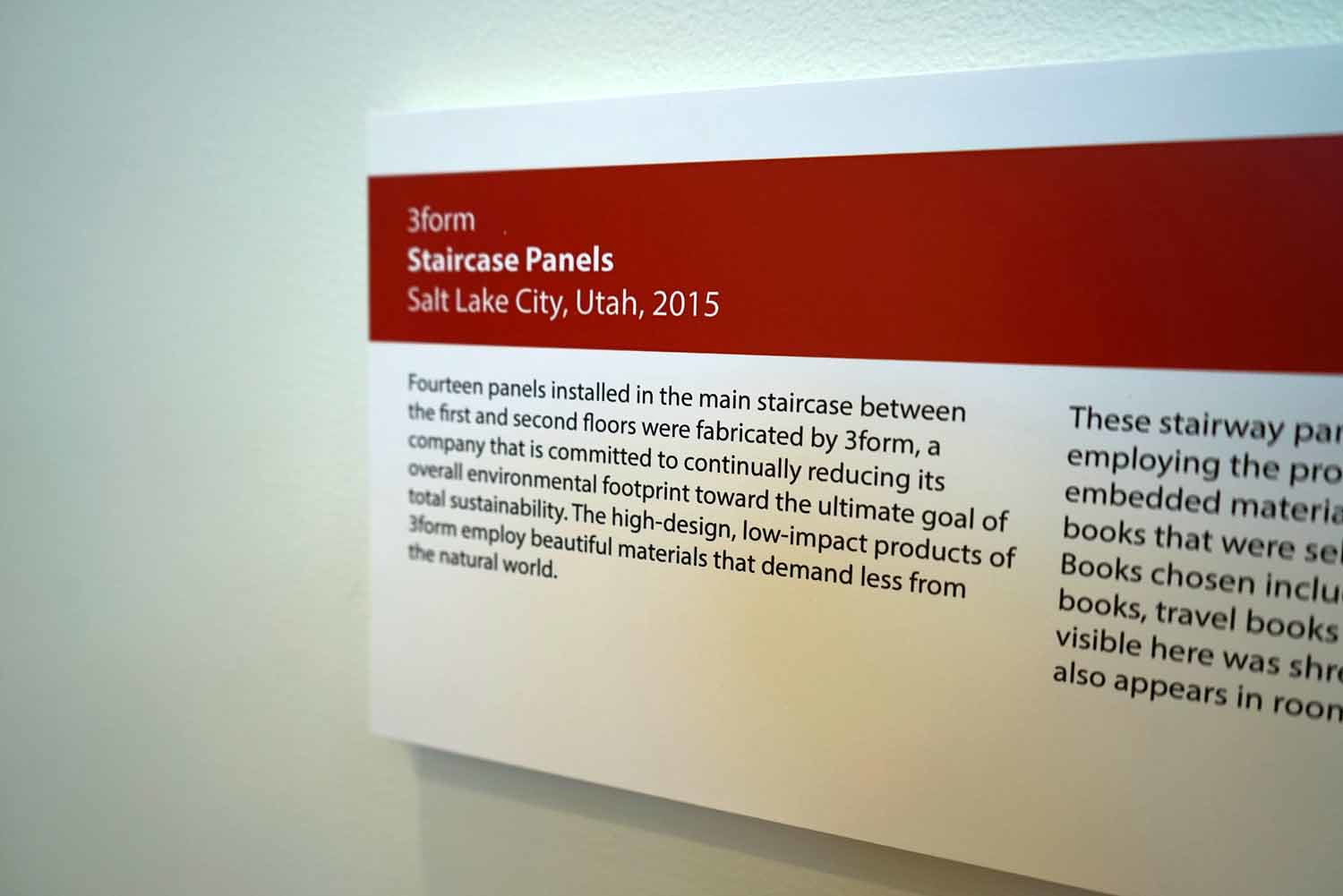The image depicts a descriptive plaque, likely from a museum exhibit, mounted on a white wall. The plaque is rectangular, oriented horizontally longer than vertically, and features a white background with a prominent red band at the top. In the red band, there is white text that reads, "Three Form, Staircase Panels, Salt Lake City, Utah, 2015." Below this band, the background is white and the text is in black. The readable text on the left side of the plaque states: "Fourteen panels installed in the main staircase between the first and second floors were fabricated by Three Form, a company committed to continually reducing its overall environmental footprint towards the ultimate goal of total sustainability. The high-design, low-impact products of Three Form employ beautiful materials that demand less from the natural world." The right side of the text is cut off and partially visible, starting with, "The stairway," but the rest of the sentence is unclear. The photograph of the plaque appears to be cropped, omitting some parts of the text and revealing part of the wall it is mounted on.